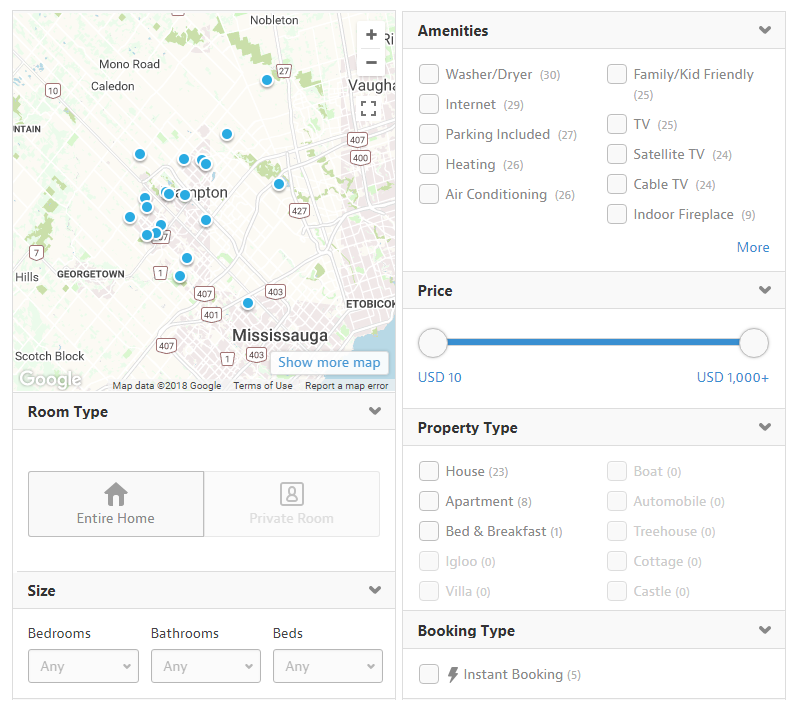The provided image is a screenshot from a third-party booking search site specifically tailored for home or general rentals. The screenshot is divided into two sections:

**Left Section:**
- **Top**: Dominated by a large Google map populated with numerous location pins indicating the available properties.
- **Below Map**: 
  - A grey drop-down box labeled "Room Type" with an arrow indicating the option to select; it currently shows “Entire Home” and “Private Room” as selectable options, with "Entire Home" being chosen.
  - **Size Category**: Includes a drop-down menu allowing for the specification of size-related parameters which encompass "Bedrooms," "Bathrooms," and "Beds." All these options are presently set to "Any."

**Right Section:**
- **Category: Amenities**: 
  - Numerous amenities are listed with checkboxes. For example, a checkbox next to "Washer and Dryer" followed by a parenthetical indicating the number of listings offering this feature.
- **Price Category**:
  - Features a drop-down menu and a slider bar below it, allowing users to set a minimum and maximum price range for their rental search.
- **Property Type**:
  - Displayed in two columns, each property type has a checkbox. For instance, "House" is listed with a parenthetical (23), indicating the number of houses available.
- **Booking Type**:
  - This includes a drop-down menu labeled "Instant Booking" with a parenthetical (5) indicating the number of properties that are available for instant booking.

This detailed layout provides an organized interface for users to refine their rental property search according to various criteria including room type, size, amenities, price, property type, and booking type.